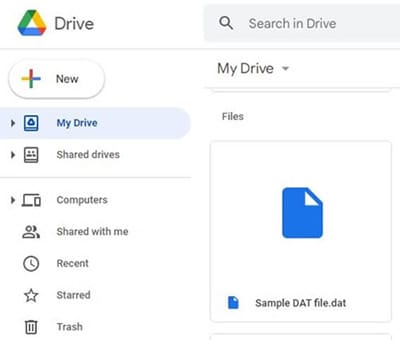The image features a screenshot of Google Drive's main interface. In the upper left-hand corner, the iconic Google Drive logo is prominently displayed. The logo is triangular and composed of green, yellow, blue, and a small touch of red colors. To the immediate right of the logo is the word "Drive" in clean, readable text. On the upper right-hand side, there is a search bar labeled "Search in Drive."

Beneath the top navigation, the interface is divided into two main sections. The left section serves as a menu, while the right section displays the contents based on the selection from the menu. At the top of the left menu, there is a white button labeled "New," featuring a Google-themed colored plus sign. Directly below this is the "My Drive" menu, which is currently the selected option.

On the right side, aligned with the "My Drive" selection, "My Drive" is displayed at the top of this section with a drop-down arrow beside it. The interface is divided by two gray separator bars. Below these bars is a labeled box titled "Files," and within this box, there is a sample file named "file.docx" prominently shown.